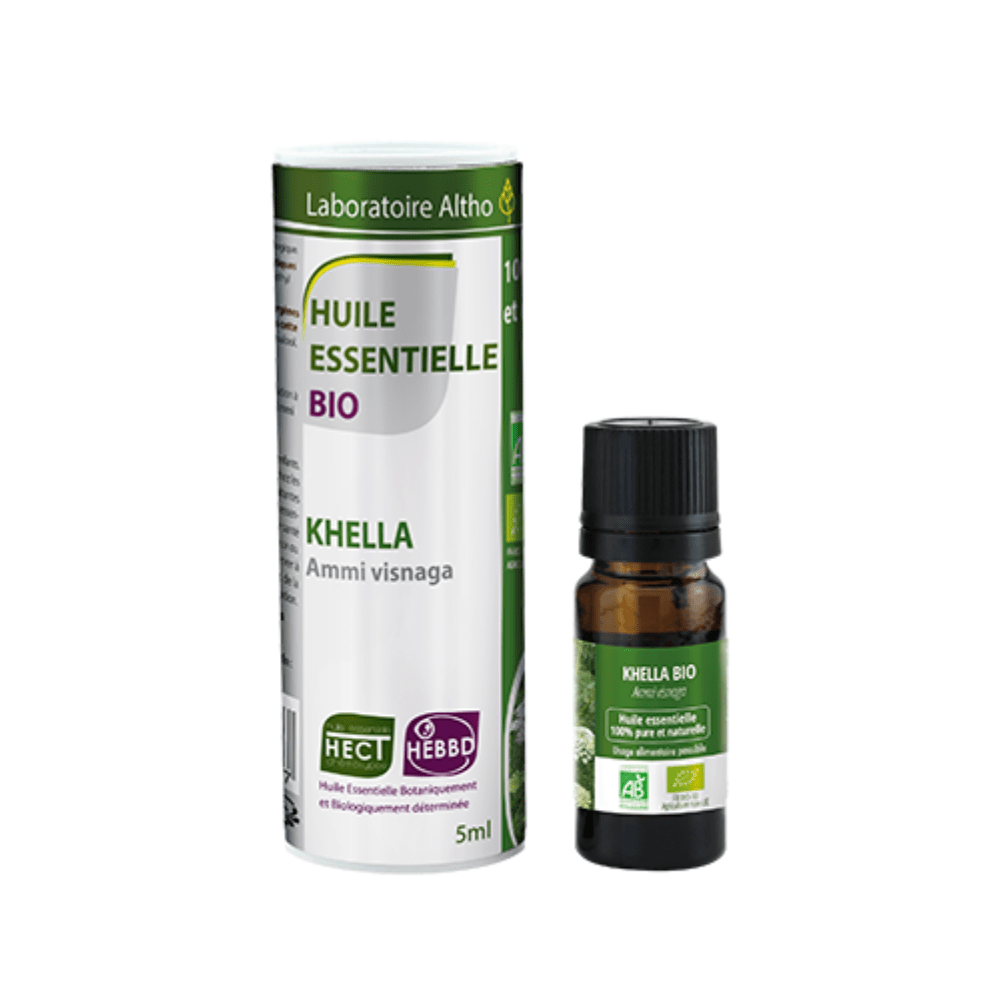The image depicts a beautifully arranged product advertisement display against a stark white background. On the left side of the image, there is a tall, cylindrical canister reminiscent of a Pringles container, adorned with a plastic round lid. This canister is primarily white with accents of green and gray and features detailed text in what appears to be French. The label at the top includes a yellow leaf emblem and reads "Laboratoire Altho." Below this, the white area with a gray leaf icon states "Huile Essentielle Bio" in purple text, followed by "Khella Ammi Visnaga."

To the right of the canister, there's a smaller bottle that looks like it could contain essential oil. This bottle has a black cap and a green label with white text that reads "Khella Bio," which is spelled out as K-H-E-L-L-A, with other smaller writing beneath it. The bottle itself is dark tinted and transparent, offering a sophisticated contrast to the larger container. The overall setting is minimalist, with the products standing out prominently against the empty whiteness, emphasizing their sleek design and potentially medicinal or beauty-oriented purpose.